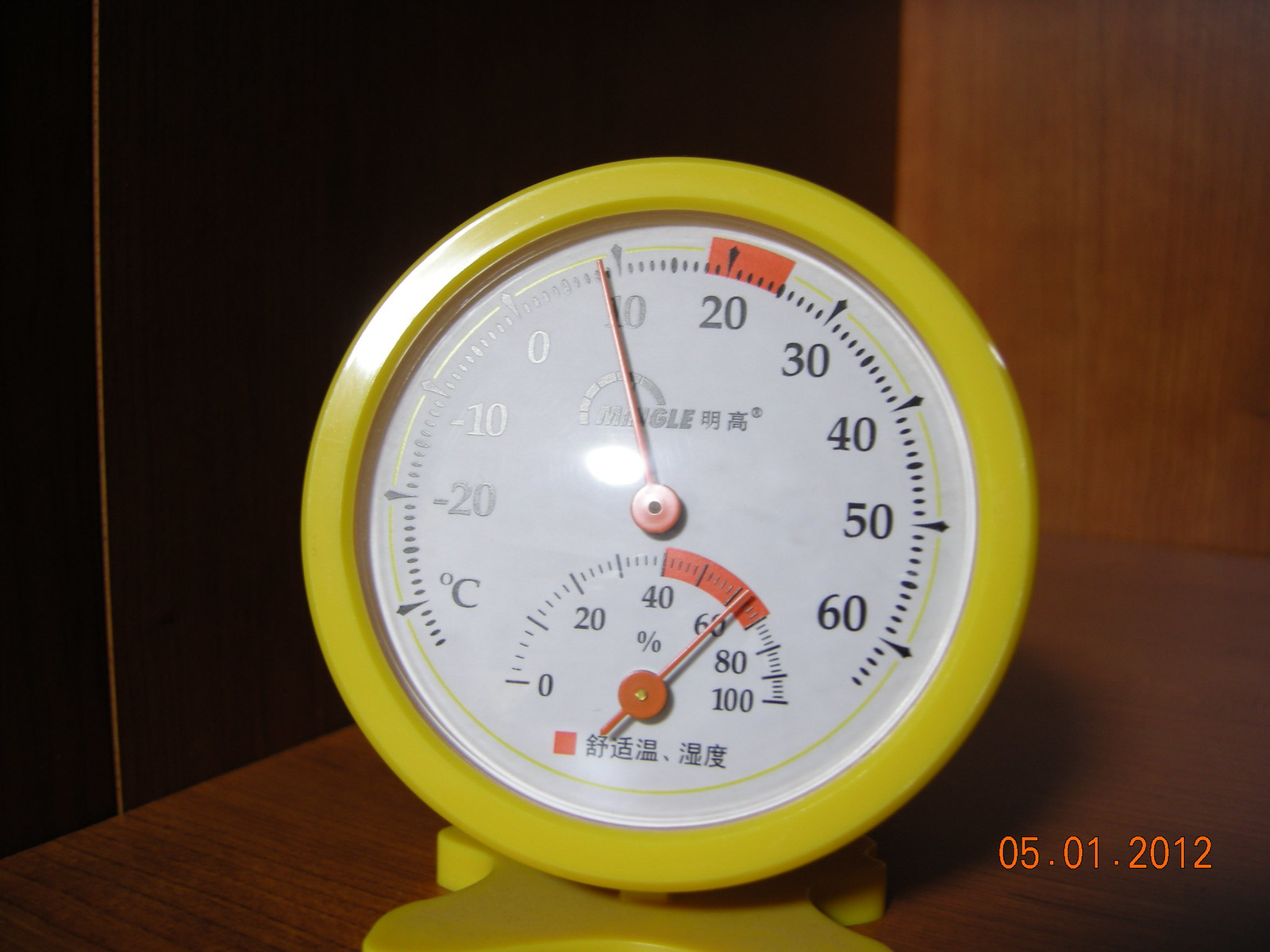A functional and basic thermometer-hygrometer combination device, predominantly designed for utility rather than aesthetics, is depicted against a backdrop that appears to be a wooden bookshelf. This clinical-looking instrument measures both air temperature and humidity, with clear, precise markings. 

The temperature dial ranges from -20 to +60 degrees Celsius, with a red-highlighted section from approximately 18 to 25 degrees Celsius, indicating a warmer range. A single needle points to the current temperature.

Below the temperature dial, there is a smaller semicircular gauge marked from 0 to 100 percent, displaying humidity levels. A red warning section spans from 40 to 60 percent humidity, suggesting a critical range. The device also features Chinese characters at the bottom.

The photograph is date-stamped as January 5, 2012.